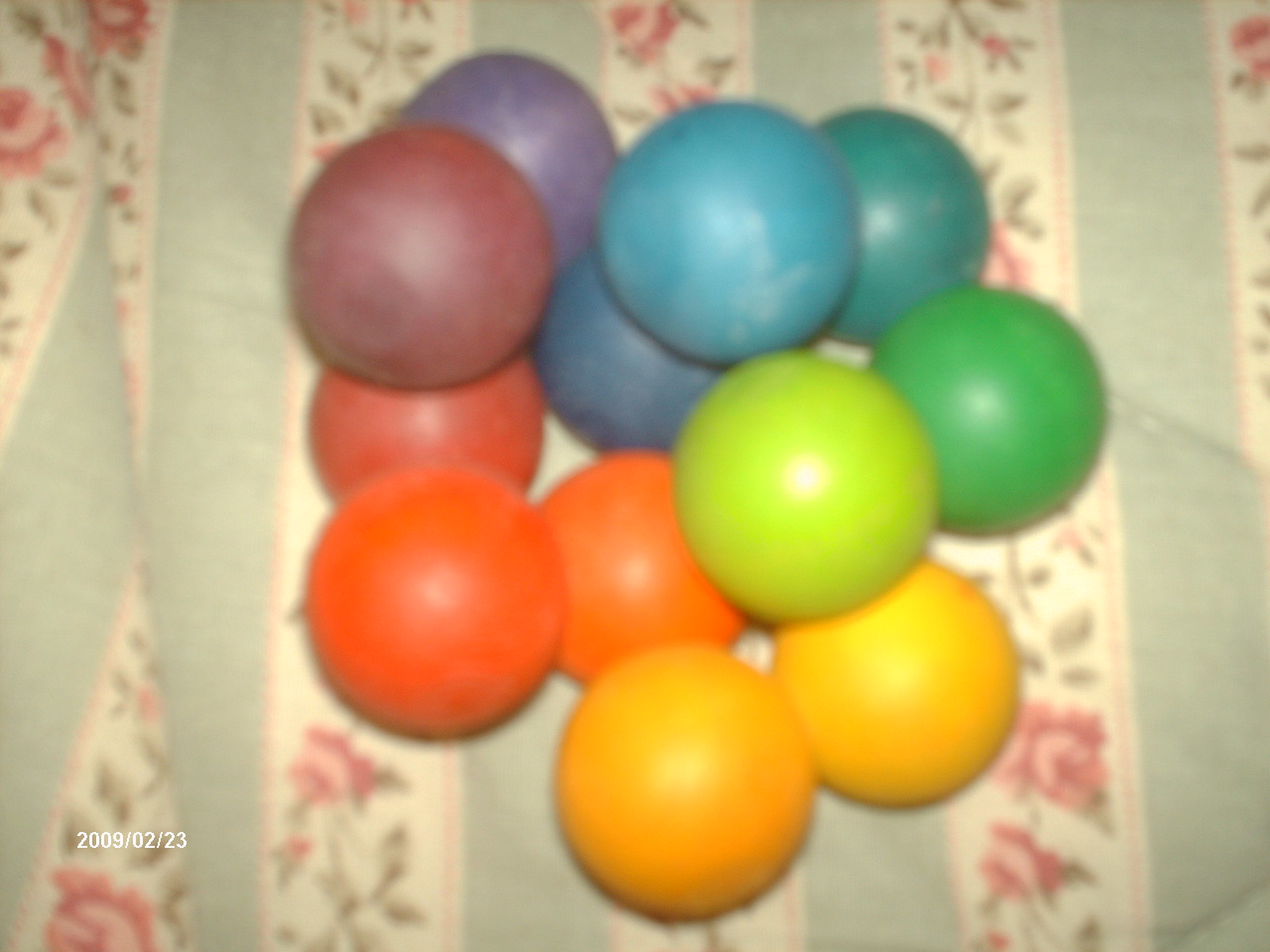The slightly out-of-focus color photograph, dated 2009-02-23, captures an assortment of twelve small, colorful rubber balls piled on a striped cloth. The cloth features alternating bands of light blue and white, adorned with pink roses and green leaves on the cream-colored stripes. The balls are in various vibrant shades: two light orange, two medium-shade orange, one red, two blue, one teal, one purple, one grayish-purple, one dark green, and one light green. The majority of the balls are nestled on the fabric, with three situated on top of the others. The overall arrangement and the cloth prevent the balls from rolling away, creating a visually captivating and colorful composition.